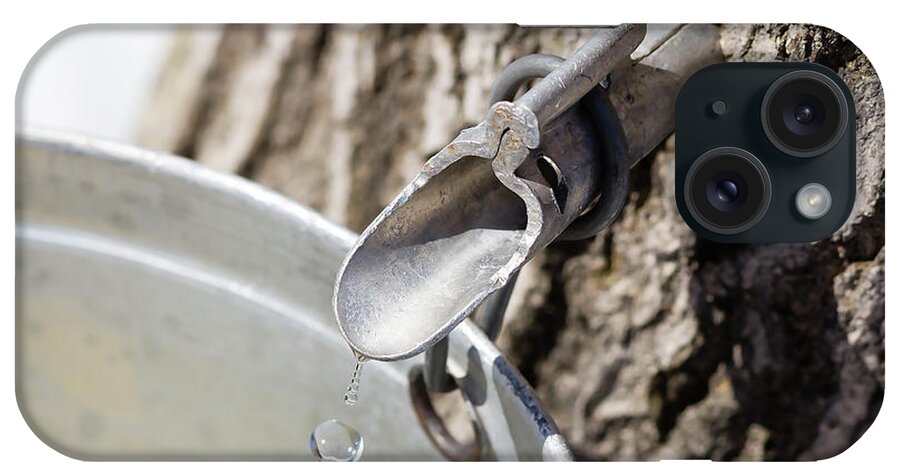This image, printed on the back of a dark grey cell phone case, showcases the process of sap extraction from a tree. The phone, oriented on its side, displays two cameras in the right corner, all within the rounded rectangle shape of the case. The visual focuses on a dull silver metal spigot, attached to a tree trunk with rough, textured bark, from which sap drips steadily. Below the spigot, a matching silver metal bucket catches the sap, with one large drop about to fall into it. The scene is detailed with shadows suggesting a sunny day, adding depth to the photo-realistic or possibly photoshopped rendering on the case.